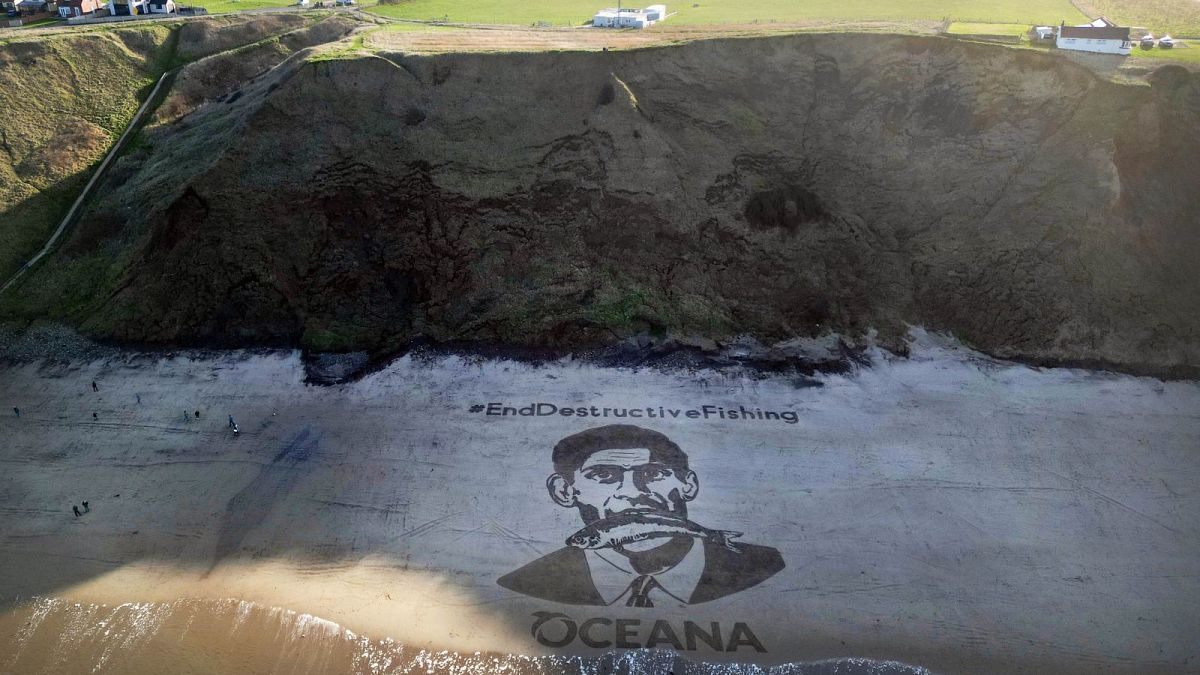The photograph captures a striking political message projected or painted on a beach below a towering rocky hill. The massive image spans from the base of the hill all the way to the shoreline, occupying the central section of the photograph. Rendered entirely in black and white, the artwork features a man in a suit holding a whole fish in his mouth, accompanied by the text “#IndestructiveFishing” and “Oceana” at the bottom, suggesting a critique of harmful fishing practices. The sand in this area appears stark white, contrasting sharply with the natural brown hue of the surrounding sand, which is highlighted by the crashing waves of brownish water in the lower left corner. Small figures—people, likely beachgoers—are visible walking near the illuminated water. The background reveals lush farmland with green grass and scattered farmhouses up on the cliffs to the far upper left and right of the image. The photo, seemingly taken from a high vantage point, like a drone or helicopter, emphasizes the imposing size of the protest art against the serene coastal landscape and nearby homes.